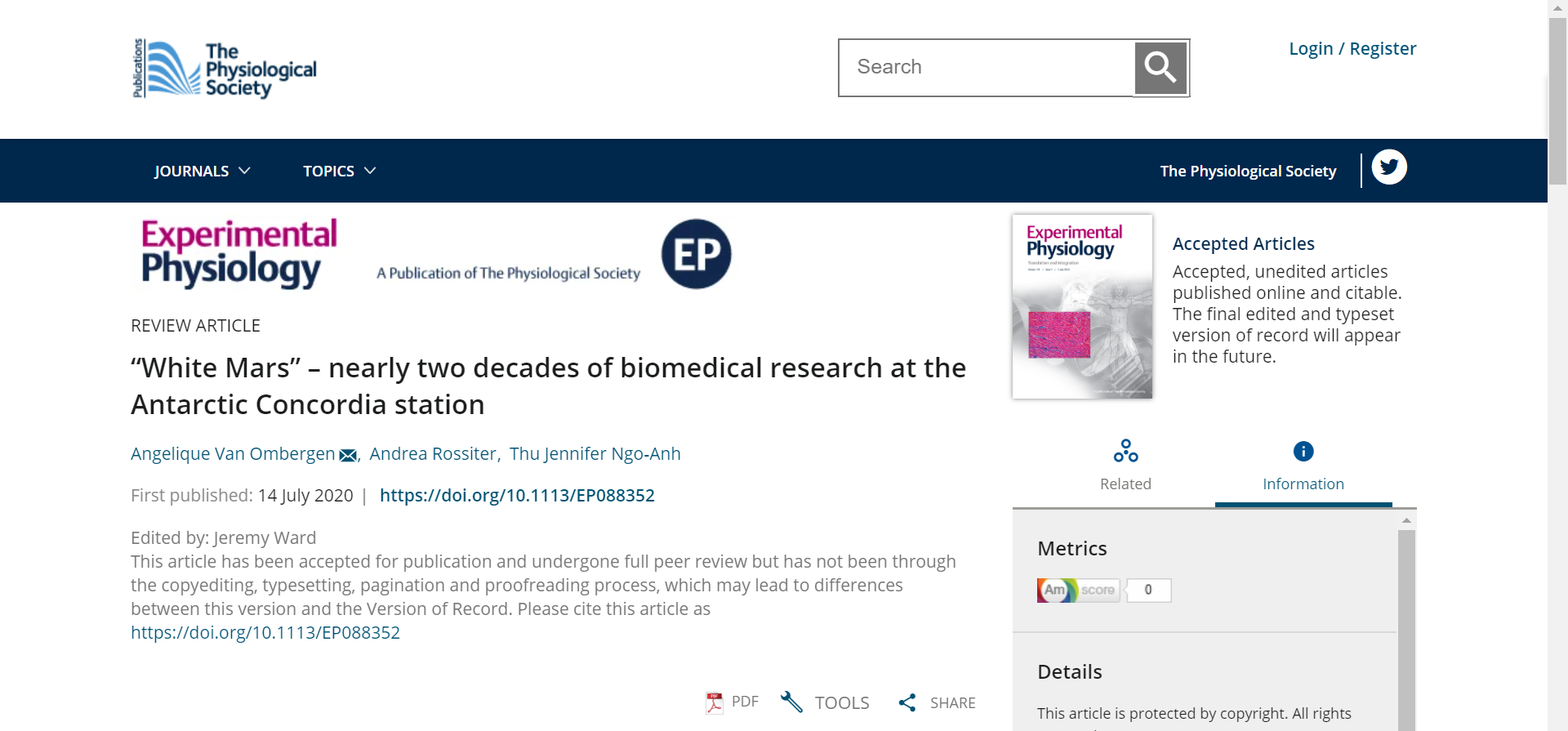On this image, the page has a clean, white background. At the top left, it prominently displays the title "The Psychological Society Publications" in black text accompanied by an icon with blue accents. Centrally at the top, there's a grey search bar, while the top-right corner features two blue buttons labeled "Login" and "Register."

Just below, the header of the website boasts a purple background, containing navigation tabs such as "Journals," "Topics," "The Psychology Society," and a Twitter icon, all in white text. Continuing downward, the background reverts to white, where the heading “Experimental Psychology” is displayed in bold pink and blue text. 

The subtitle "A Publication of Psychological Society EP" is noted, along with the article type “Review Article.” The main content section starts with a synopsis stating, "White mass nearly two decades of biomedical research at the Antarctic Concordia Station," attributed to authors Angelico van Oombergen, Andrea Rosita, and Du Chenyifango, whose names are in blue. It signifies that the article was first published on 14 July 2020, and edited by Jeremy Ward.

A disclaimer follows, indicating that the article, though accepted for publication, is still subject to the copy-editing, typesetting, pagination, and proofreading processes, potentially leading to differences between this version and the final version. The text reminds readers to cite the article using a DOI URL, which is also listed in blue.

At the bottom of the page, there are icons for a PDF download, tools, and sharing options. On the right side, there's a book cover titled "Experimental Physiology," introducing an accepted and edited article that has been published online and is citable, with a final typeset version to appear in the future.

Beneath this, there are tabs for additional content like "Related Information," which includes "Matrix AM Score" and "Detail." A copyright notice indicates that this article is protected by copyright and clarifies that the journal's name is "Experimental Physiology," not "Psychology." At the top, it is further specified that it belongs to "The Physiological Society."